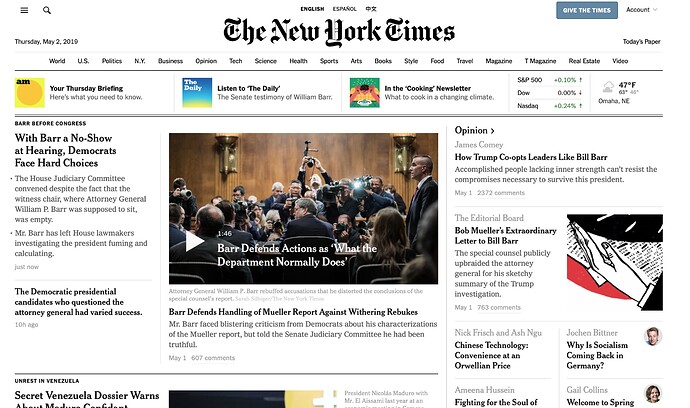This screenshot captures a New York Times article viewed in landscape mode on May 2nd, 2019. The interface identifies the publication's English version in the upper center, confirming the date as Thursday, May 2, 2019, in the upper left corner. The upper right corner displays a "Give the Times" button, indicating a subscription to the New York Times.

The primary headline on the left reads: "With Barr a no-show at hearing, Democrats faced hard choices." Below, it mentions that Democratic presidential candidates questioning the Attorney General achieved varied levels of success. On the right side, another headline states: "Barr defends actions as what the department normally does," with a subheading noting "Barr defends handling of Mueller report against withering rebukes."

Further down on the right, an opinion piece by someone named James discusses "how Trump co-opts leaders like Bill Barr," although the name is partly obscured due to gray text against a white background. Another partially readable section below mentions "Bob Mueller's extraordinary letter to Bill Barr."

Additional topics appear at the bottom, including "Chinese technology, convenience at an Orwellian price" and "Why is socialism coming back in Germany." In the bottom left corner, there is a heading about unrest in Venezuela, specifically a "secret Venezuela dossier," although this is cut off and not fully visible, indicating that the screenshot was taken while scrolling through the page.

Overall, the screenshot seems to focus on various content related to Attorney General Bill Barr, Mueller's report, and other contemporary issues.